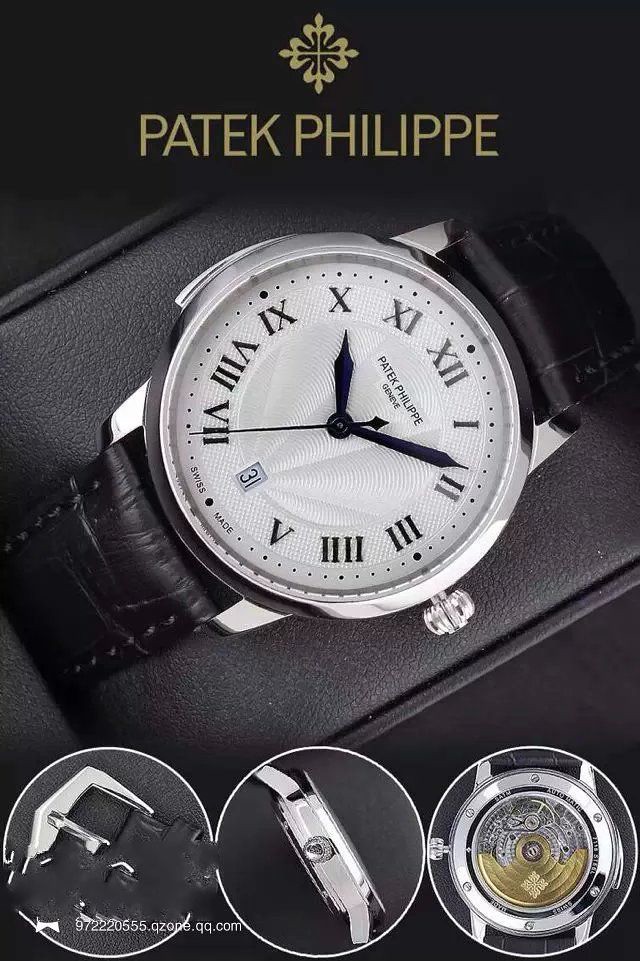This advertisement for a Patek Philippe men's wristwatch is set against a sleek black background. At the top, elegant gold capital letters spell out "PATEK PHILIPPE," accompanied by a distinctive diamond design above. 

The main focus of the image is a close-up of the wristwatch encased in a sophisticated black case. The watch itself features a polished stainless steel case, with a small silver wind-up button on the side. The watch face is pristine white, adorned with classic black Roman numerals. The black minute, hour, and second hands gracefully sweep across the dial. Prominently displayed at the top of the watch face is the Patek Philippe logo in black. At the lower part of the dial, where the number 6 would typically be, there is a small window showcasing the date, which is set to the 31st. 

Below the image of the watch, three small white circles highlight intricate components of the watch, emphasizing its craftsmanship and attention to detail. This sophisticated layout elegantly underscores the luxury and precision associated with the Patek Philippe brand.